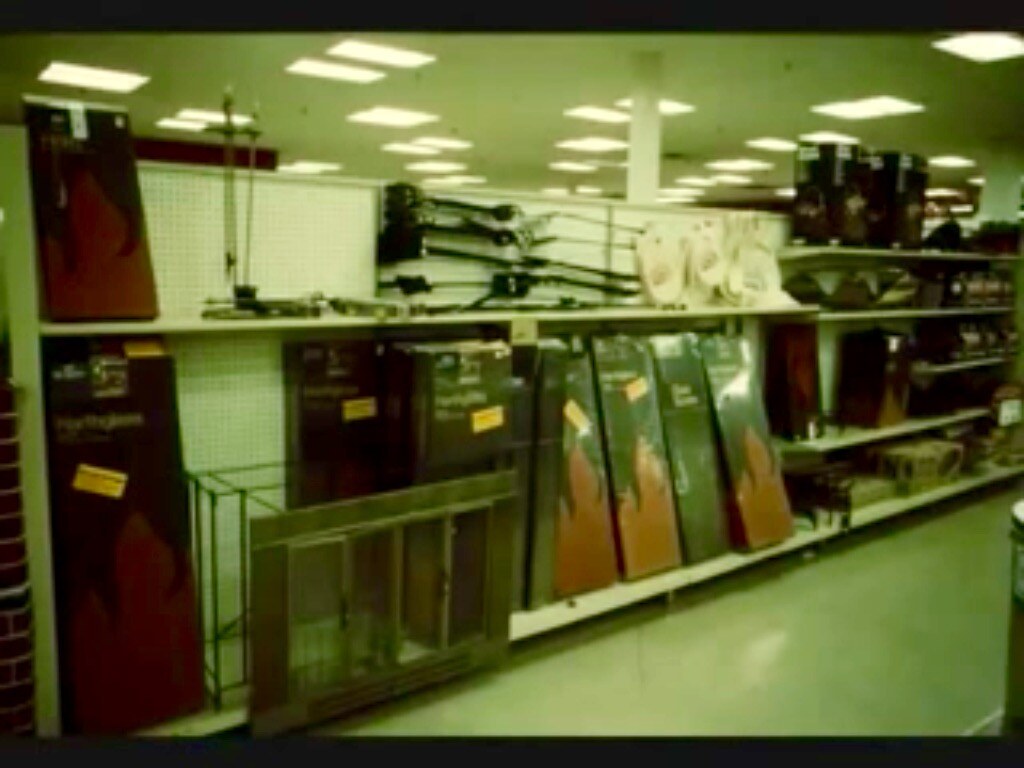The image captures an aisle inside a well-lit store, specifically dedicated to home essentials. The floor is polished and off-white, reflecting the bright light emanating from the numerous square-shaped ceiling lights that uniformly cover the entire ceiling. The shelf in focus is stocked with various items, one of which is a distinguishable red box, although the text on it is blurred and unreadable. Off to the left-hand corner of the image, there appears to be a section of a brick-patterned wall, adding an element of rustic design to the store's interior.